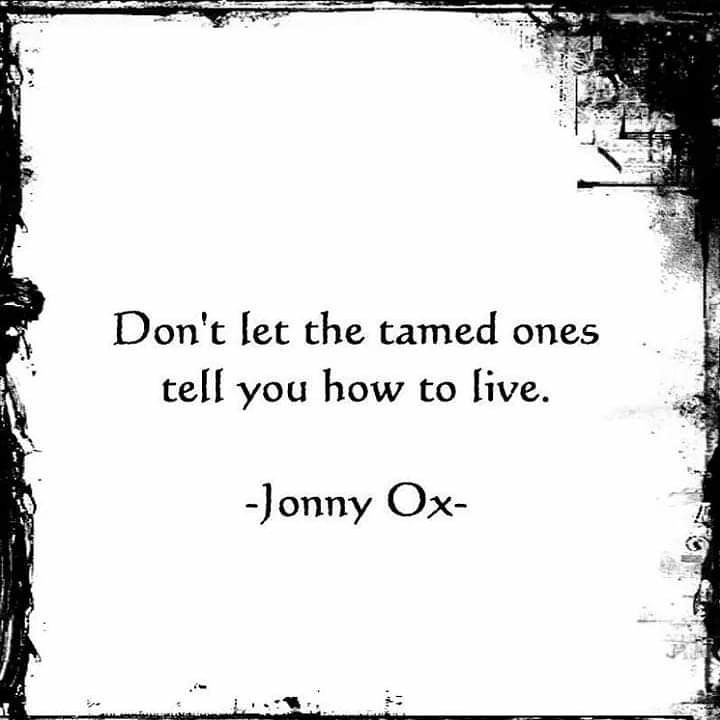The image is a black and white square with irregular black patterns resembling paint splotches around the border, with a notable blacked-out area in the upper right corner and some gray shades towards the center. The black borders appear as if the ink is slightly faded into the white center, creating a printwork effect. In the very center, the image prominently features the black-printed inspirational quote: "don't let the tamed ones tell you how to live." Below this quote, the name "Johnny Ox" is printed, framed by dashes on either side. The name "Johnny" is specifically spelled "J-O-N-N-Y." The left side of the border has a pattern that might visually resemble a person's head leaning forward, but this could also be an optical illusion created by the random spread of the black ink. This stylized image evokes a sense of artistic texture, typical of inspirational quotes found on social media platforms like Pinterest.